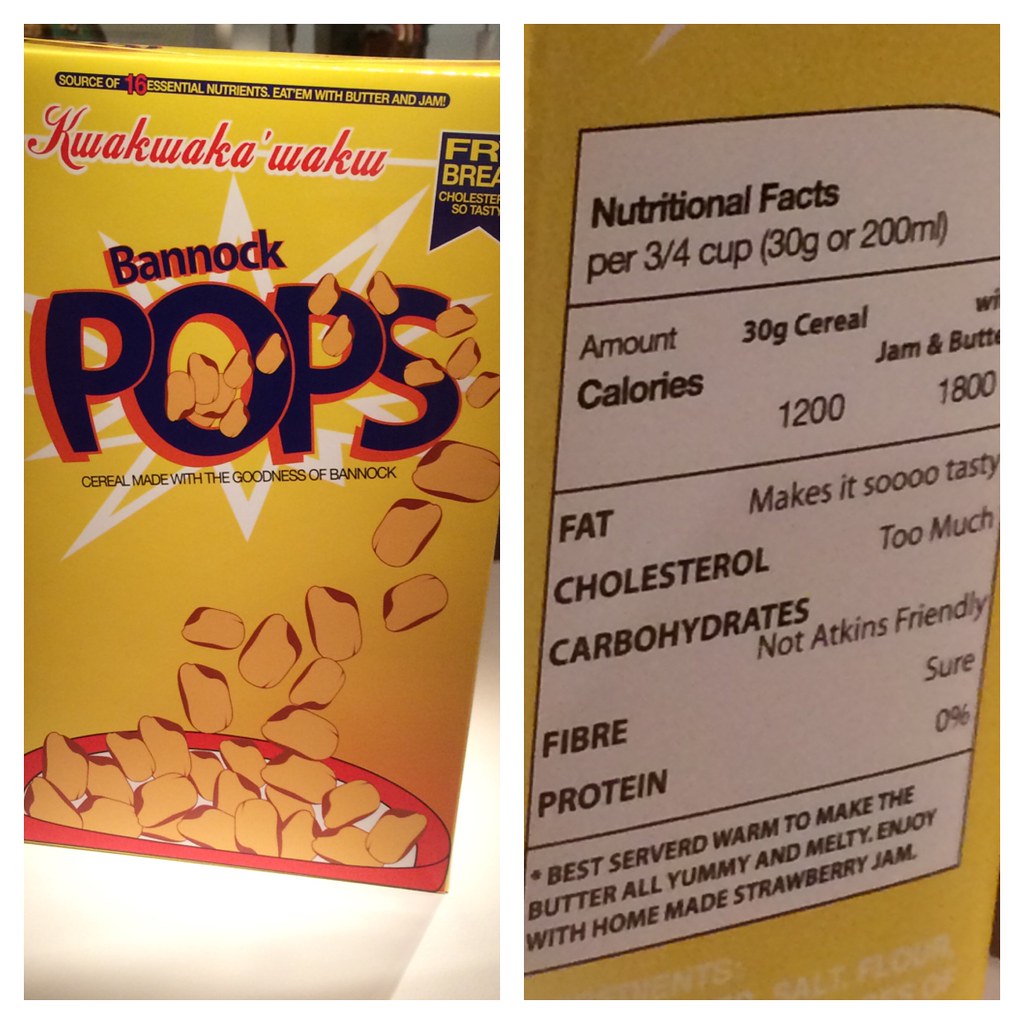The image is split into two sections depicting two different food products. 

On the left side, a brightly colored yellow cardboard box labeled "Bannock Box" is prominently featured. This box showcases a cereal made with the wholesome goodness of Bannock. The packaging is visually engaging with rectangular cereal pieces illustrated as popping out from the box, creating a dynamic visual effect. Within a star-shaped graphic that has a blue and red border inside a white star, these cereal pieces appear to cascade into a white bowl with a red rim.

The right side of the image highlights the back of another product's packaging, which is also yellow but clearly different from the Bannock Box. This section provides detailed nutritional information for a serving size of three-quarters of a cup (30 grams) or 200 milliliters. The table lists the calorific content, fat, cholesterol, carbohydrates, fiber, and protein. Additionally, this packaging includes a serving suggestion, recommending that the product is best enjoyed warm to allow the butter to melt into it deliciously, and pairs well with homemade strawberry jam.